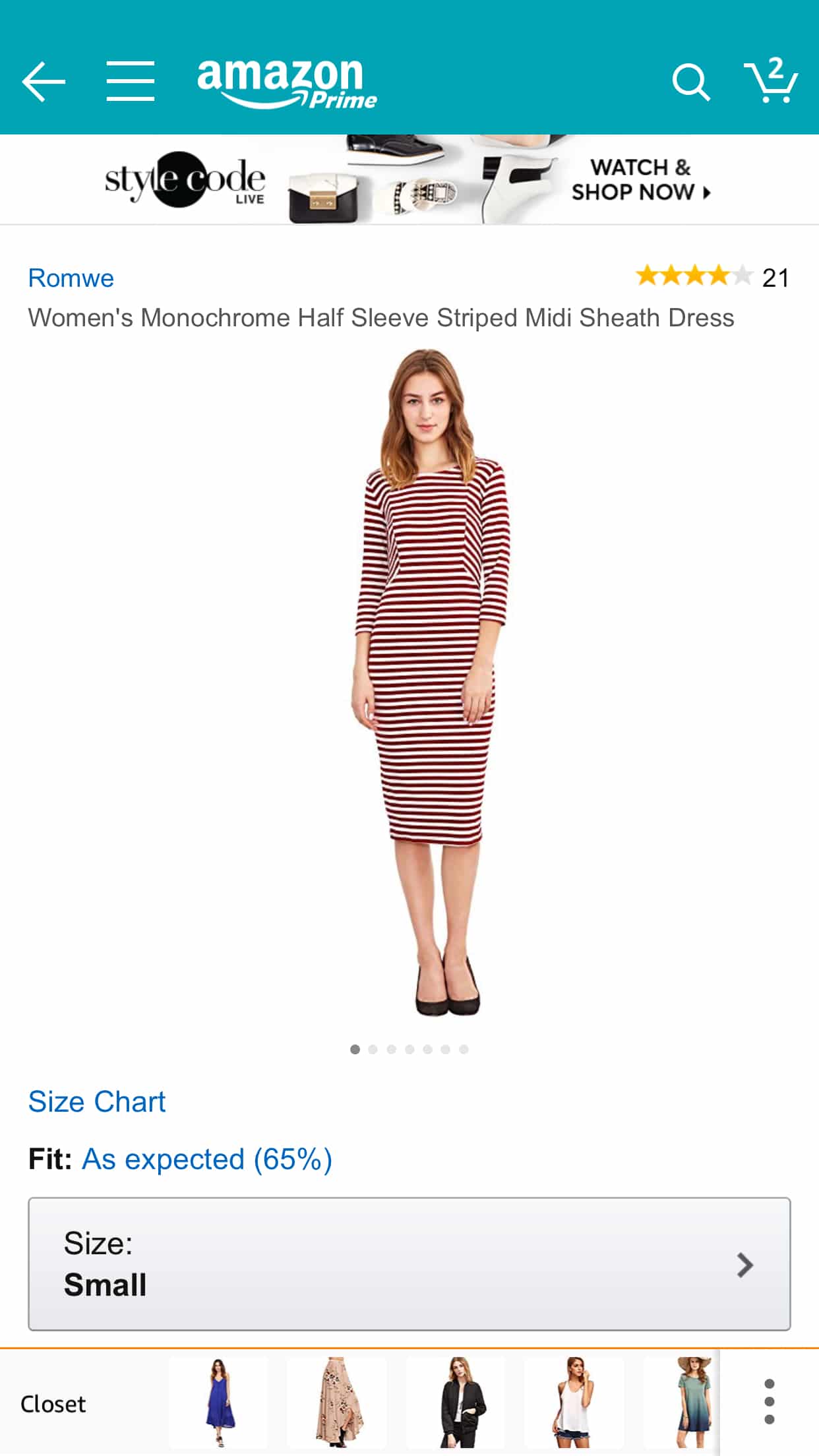This screenshot features a webpage from Amazon Prime with a teal-colored header. The header is organized with a left-pointing arrow, followed by three horizontal bars, the Amazon Prime logo, a search magnifying glass icon, and a shopping cart icon with the number two indicating items inside it.

Directly below the header, there's an ad banner for Style Code Live, a fashion-oriented segment, which includes options to "Watch" and "Shop Now." Beneath this banner is a product page for an article of clothing from ROMWE. The product title is displayed in blue text as "ROMWE," followed by "Women's Monochrome Half-Sleeve Striped Midi Sheath Dress" in black text. The dress has received a rating of 4 out of 5 stars based on 21 customer ratings.

The main image on the product page shows a slender, brunette woman in her twenties with shoulder-length wavy hair wearing the striped dress. The dress extends past her knees, and she pairs it with black shoes. Below the product description, a size chart indicates that the item fits as expected 65% of the time. There is also a button displaying the size "Small."

Further down, there's a section labeled "closet," showcasing approximately five images of various clothing items worn by different models.